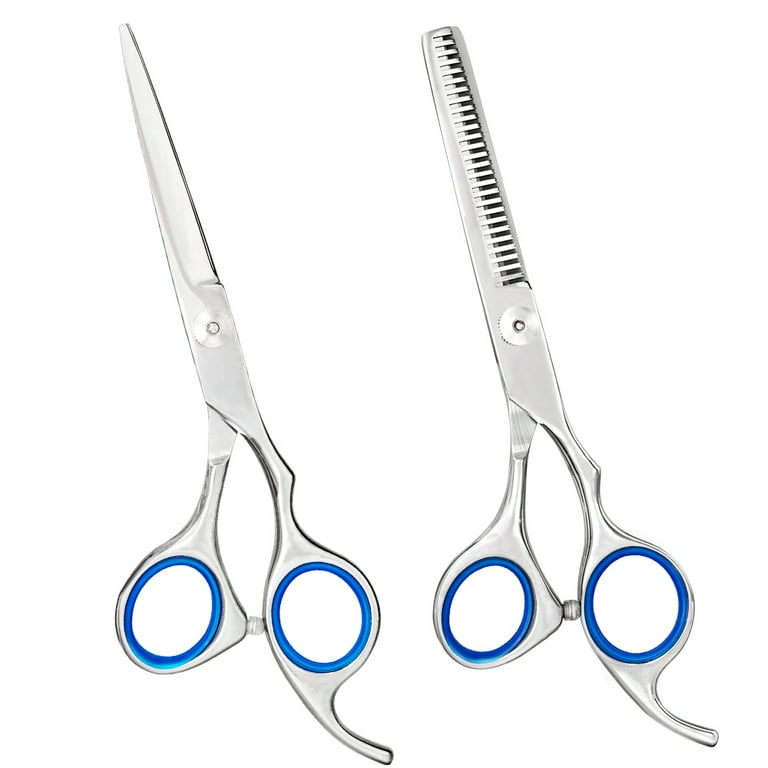The image is a full-color photograph featuring two pairs of metallic silver scissors, set against a stark white background with no additional shapes or borders. Both pairs of scissors have blue trim around the finger holes. The scissors are positioned with their handles at the bottom and their blades angled upward and to the left. The pair on the left is a traditional design with two flat blades that meet at a pointed tip. The pair on the right is specifically for haircutting, characterized by one blade with rectangular teeth, resembling a comb, and the other a standard blade. Both pairs share the same blue-ringed handles and sleek silver finish, highlighting their simple yet functional design.